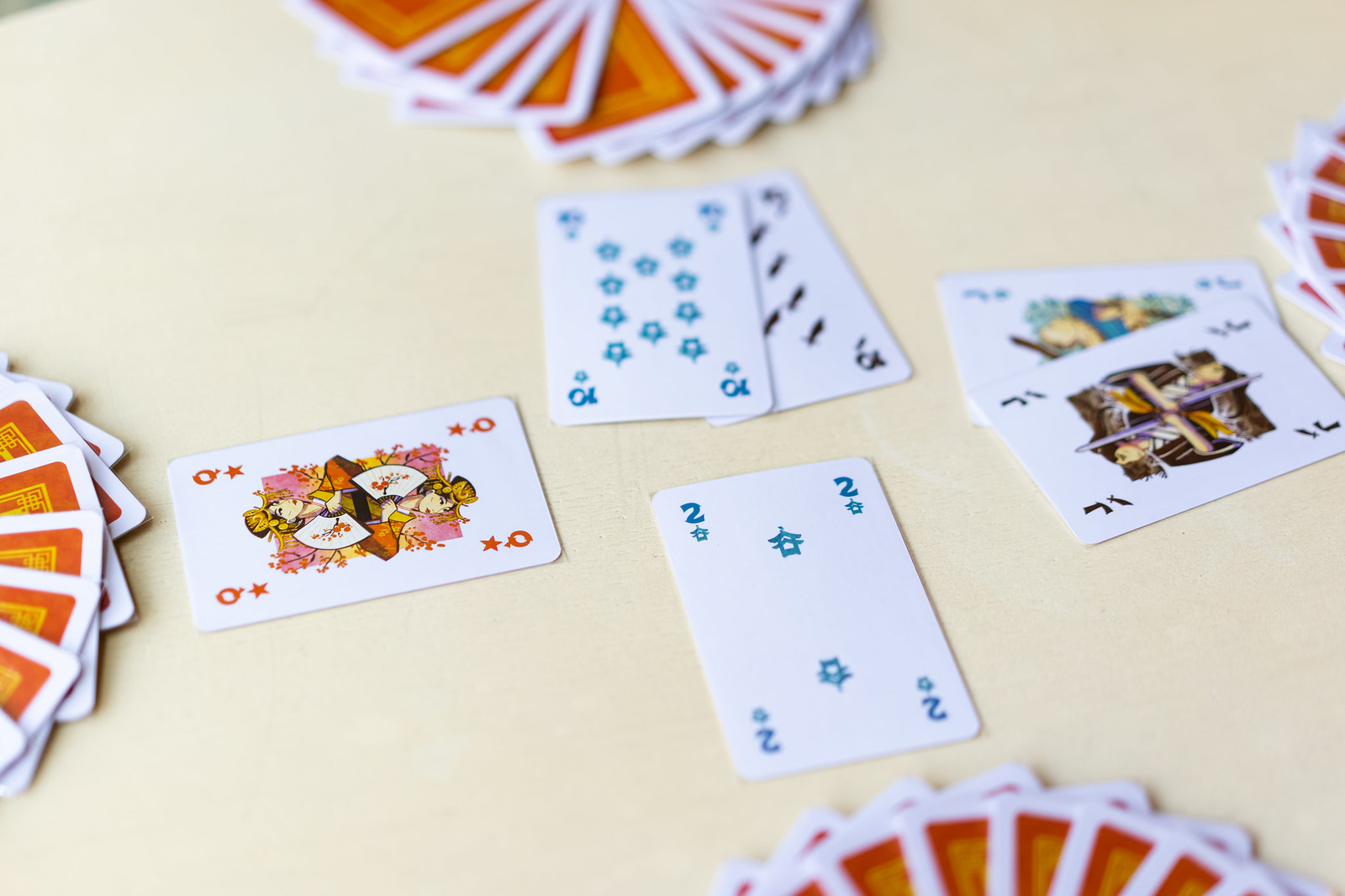This photograph captures a close-up view of a beautifully set tabletop covered with a cream-colored tablecloth that has a subtle pink tinge. The focus is on a card game with four hands of playing cards laid out in a fan-like arrangement. The cards have intricate red backs adorned with gold patterns and a classic white border. 

Each hand shows only the top third of the cards, except for the set at the top which reveals about half, albeit slightly blurred. In the foreground, two cards are turned face-up in both the top and right hands, while one face-up card is visible in the bottom and left hands. These face-up cards have an ornate oriental Chinese theme, featuring unique suits such as swords, suggesting that this may be a specialized deck rather than a traditional set of playing cards. The detailed composition of the cards against the pastel backdrop creates a captivating and intriguing scene, inviting viewers to ponder the game's next move.